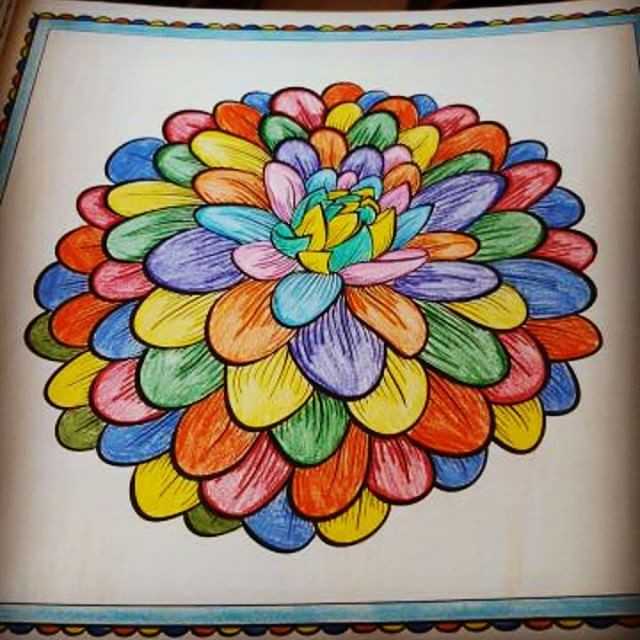A vibrant and intricate piece of artwork is seen from a birds-eye view, filling an entire white page. At the center, a rose-like flower blooms, its open petals expanding outward. Each successive layer of petals grows larger, creating numerous concentric rows that cover the page. The petals are meticulously colored in a harmonious palette, including shades of purple, orange, yellow, blue, aqua, green, red, dark green, and more yellow. Surrounding the flower, a light blue border frames the composition, with tiny petals extending beyond it, alternating in the same array of vivid colors. This detailed and colorful masterpiece showcases the artist's creativity and attention to detail.